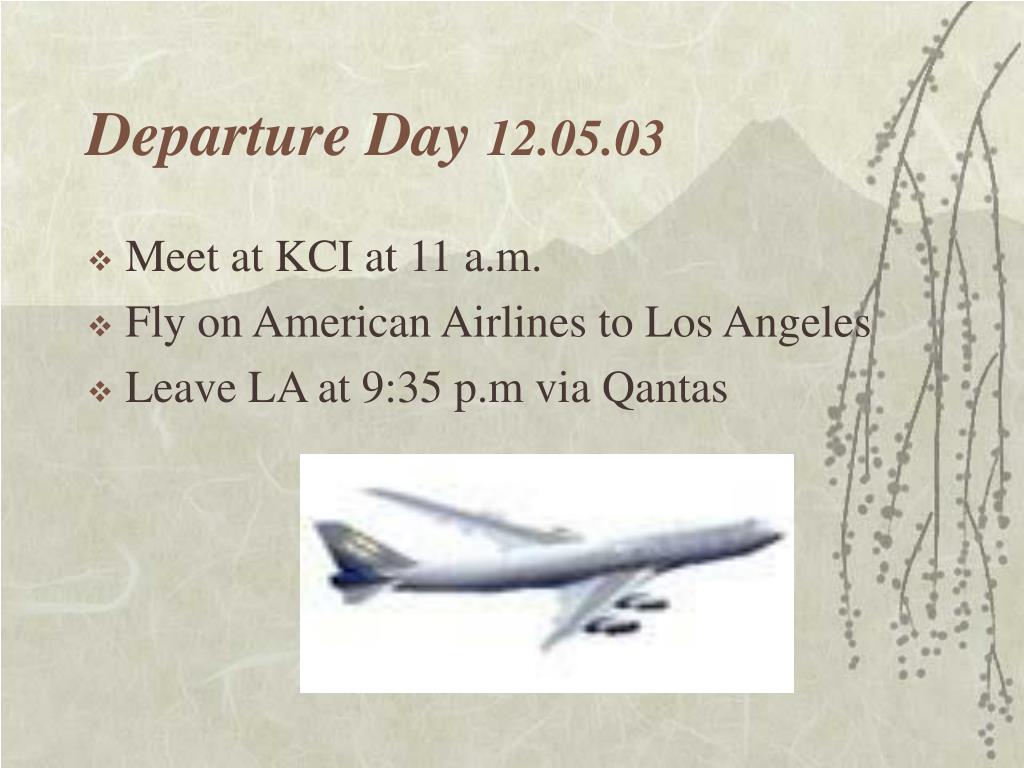The image appears to be a screenshot from a PowerPoint presentation, featuring a crinkly light beige background with pale white lines, giving it a textured appearance. On the right-hand side, a shadowy image of a mountain peak is faintly visible, accompanied by a graphic design of a tree branch with budding leaves or small circular flowers. The primary focus is on the text positioned at the top, displayed in brown fonts. The heading reads "Departure Day 12-5-03," followed by a detailed itinerary: "Meet at KCI at 11 a.m.," "Fly on American Airlines to Los Angeles," and "Leave LA at 9:35 p.m. via Qantas." At the bottom, within a horizontal white rectangle, a sideways, low-quality image of an aircraft is shown, facing right. The overall color scheme includes tan, brown, gray, white, and black.